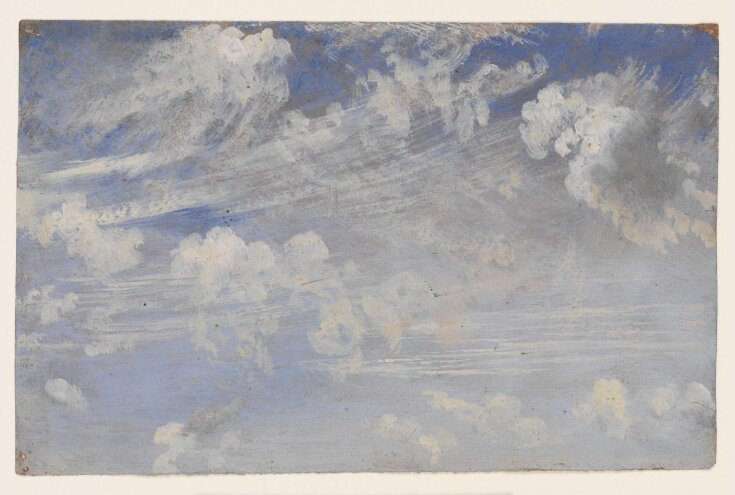This image depicts a vintage painting featuring a dynamically textured, stormy blue sky adorned with numerous clouds. The painting transitions from darker blues at the top to lighter blues at the bottom, capturing a dramatic gradient. The sky is filled with an array of clouds, painted in shades of blue, white, and light gray, giving the impression of a windy day with clouds in motion. Visible brush strokes add texture, with streaks creating a weathered, almost dry appearance. The painting is encased in a small, thick white border that adds to its rustic and antiquated charm. The brown edges of the paper further enhance its aged look, and the overall scene is accentuated by a patchy, hot modge podge effect on the surface.